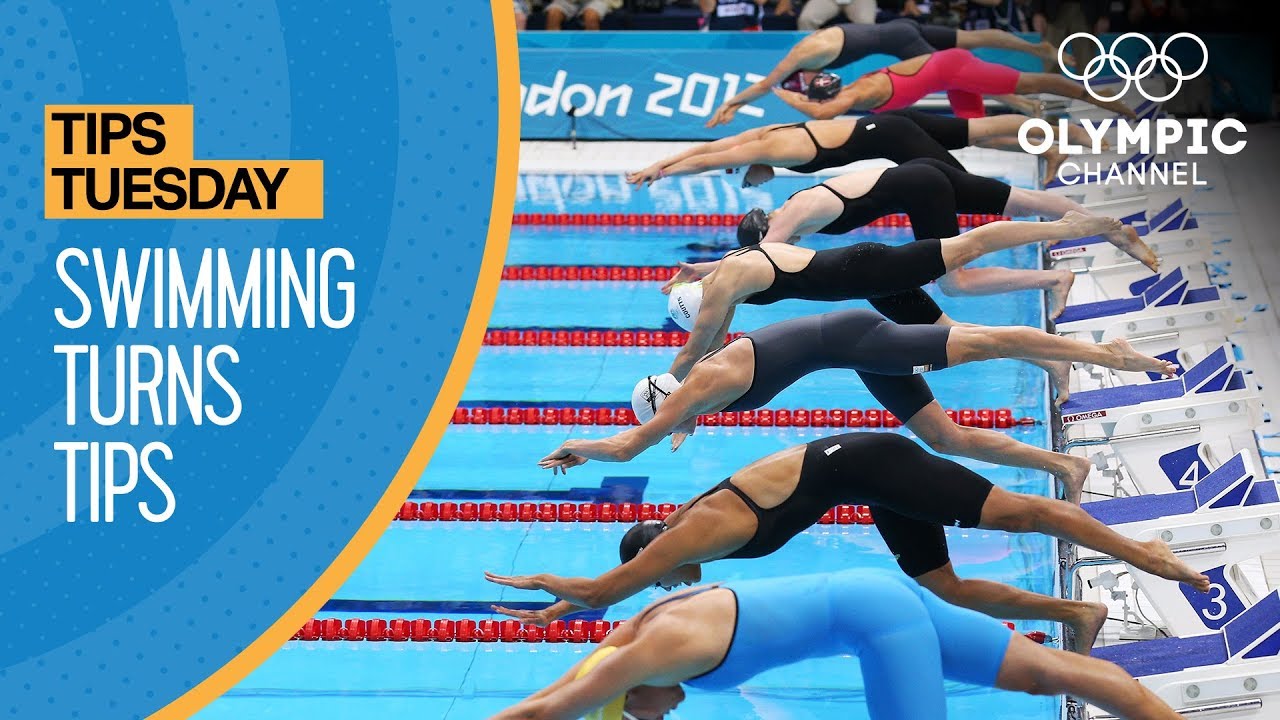The image is from the Olympic Channel, featuring eight swimmers, possibly from the London 2012 Olympics, mid-dive off of diving boards, preparing to enter the water. The swimmers are all wearing swim caps and goggles, with most donning black one-piece swimsuits, and one wearing a red suit and another blue. The upper right corner displays the Olympic Channel logo with the five white Olympic rings. On the left side, a graphic with concentric semicircles in varying shades of blue, decorated with polka dots, includes a yellow line and a yellow box that reads, in black text, "Tips Tuesday," and in white text, "Swimming Turns Tips." The image suggests a focus on techniques for turning during a swim race. Additionally, the background features red floats marking each lane.